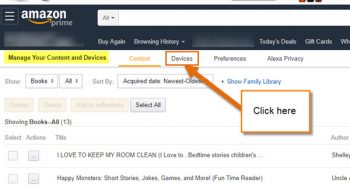A screenshot of an Amazon Prime page on a laptop. The screen displays the Amazon Prime logo prominently at the top, characterized by the white "Amazon" text and the signature orange arrow beneath, reminiscent of a Nike swoosh. To the left of the logo, there is a settings option, and to the right, a drop-down box that currently reads "All," allowing users to refine their searches.

In the navigation bar below, several options are visible including "Buy Again," "Browsing History," "Today's Deals," and "Gift Cards," with some sections blurred to protect user identity. The "Devices" option is highlighted with an orange box and an accompanying caption bubble that reads "Click Here," marked by an orange border and an arrow pointing directly to "Devices".

Beneath the main navigation, a filter is available for sorting books. Users can select genres such as "Mystery" or "Sci-Fi," and sort results by acquired date, either from newest to oldest or vice versa. Additionally, there's an option to show the family library.

Further down the page, two specific book entries are displayed. The first is "I Love to Keep My Room Clean" by Sheila, and the second is "Happy Monster Short Stories" by an author named Uncle, with the author's full name obscured.